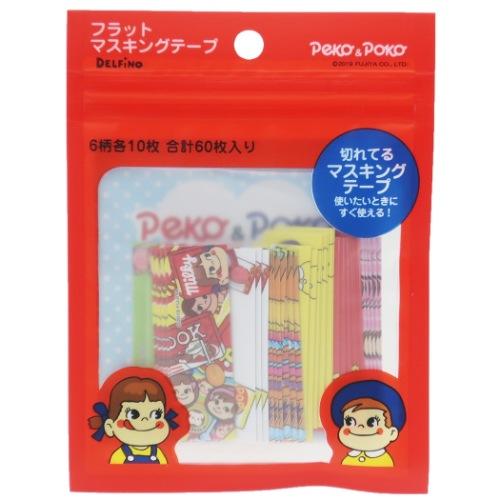A vibrant, red package, presumably of Korean origin, prominently features text that appears to be in katakana script (although this is more commonly associated with Japanese). The package includes a transparent section that offers a glimpse of its contents, which remain somewhat ambiguous, though they seem to resemble candy. The bottom portion of the packaging is adorned with photos of two children. On the left side, a young girl with pigtails tied with ribbons gazes outward, her cheeks adorned with a blush. To the right, a young boy wearing a blue hat similarly sports blushed cheeks. The playful, endearing imagery suggests the product is aimed at a younger audience, though the exact nature of the contents remains unclear.